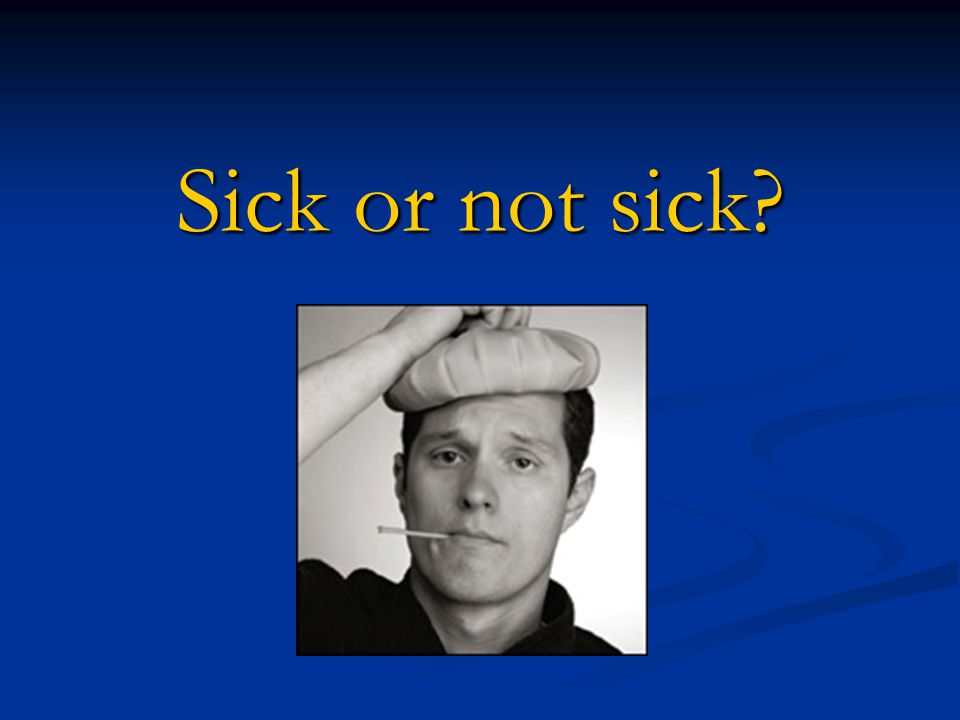The image depicts a black and white photo of a man with short dark hair and light skin complexion, wearing a short-sleeve, collared, dark-colored shirt. He appears unwell, with a thermometer in the right side of his mouth and his right hand holding an ice pack on top of his head. The man's forehead is furrowed, and his mouth is closed. The background is predominantly blue with a gradient from dark to lighter shades, featuring a subtle ripple design in the bottom right corner, possibly resembling water. Centered in the middle of the image, above the photo, in bold yellow letters, is the text "Sick or not sick?" indicating the theme of the presentation-like slide. The overall clarity and quality of the image are high, with no additional objects, people, or text present.